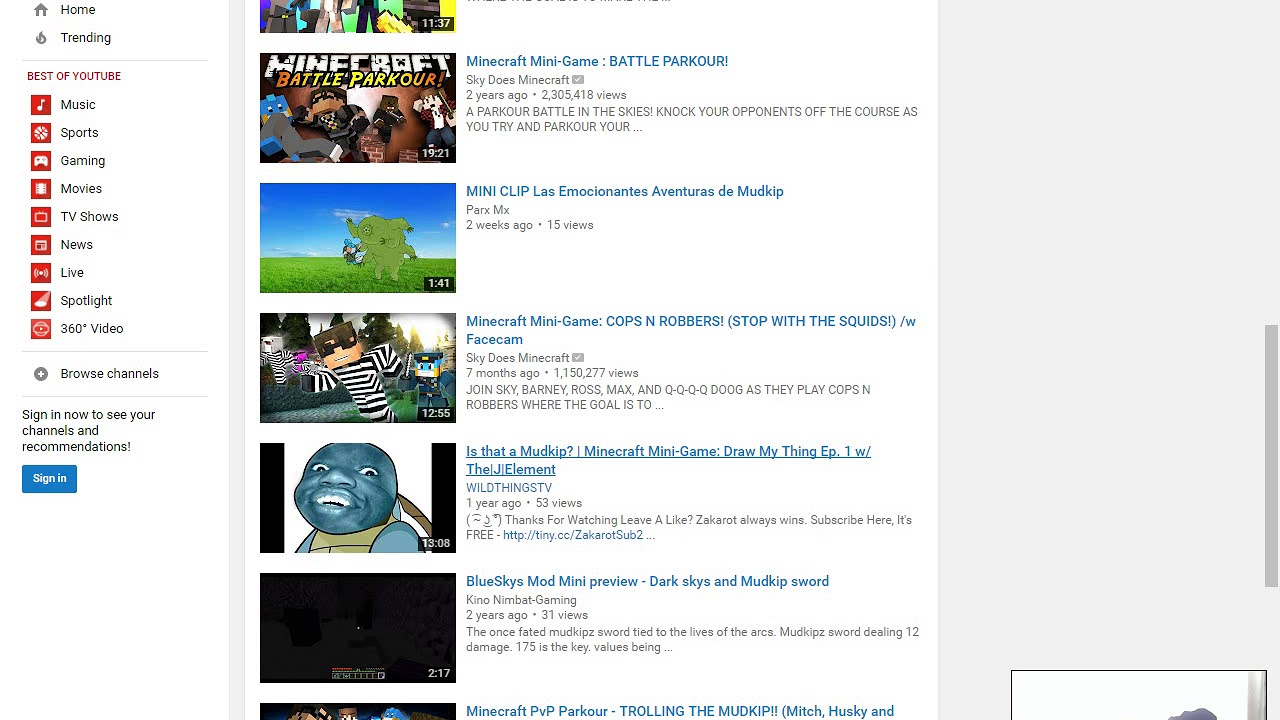A horizontally rectangular screenshot from YouTube is displayed. On the left side of the image is a vertical navigation menu set against a white background. The menu features icons and titles for different sections, starting with "Home" at the top, followed by "Trending." Below this, there's a section titled "Best of YouTube" containing various categories: Music, Sports, Gaming, Movies, TV Shows, News, Live, Spotlight, 360° Video, Browse Channels. Farther down, it prompts the user with a message: "Sign In Now to see your channels and recommendations," accompanied by a blue sign-in button.

The remainder of the image, on a light gray background, features a list of various gaming video thumbnails and titles. Each listing has a game image on the left, and to the right, detailed titles of the videos which appear to include gameplay content. They are as follows:

1. **Minecraft Mini Game Battle Parkour** - The title is partially cut off, but it suggests parkour challenges within Minecraft.
   
2. **Mini Clip** - Accompanied by a title in Spanish.

3. **Minecraft Mini Game Cops and Robbers** - Another Minecraft game mode, focused on a classic tag-and-capture style game.

4. **Stop with the Squids** - Likely a humorous or critical video involving squids in Minecraft, featuring a facecam of the player.

5. **Is That a Mudkip?** - A video possibly related to Pokémon and featuring the character Mudkip.

6. **Minecraft Mini Game Draw My Thing** - A Minecraft variant of the drawing game "Pictionary."

7. **F1, with the J element** - Potentially a reference to Formula 1 racing and a special element or feature.

8. **Blue Skies, Mod Mini Preview** - Previewing the "Blue Skies" mod in Minecraft, potentially involving new sky dimensions or weather features.

9. **Dark Skies, and Mudkip Sword** - Suggests a continuation or variant of the previous mod with additional content focused on darker skies and a special Mudkip-themed sword.

This detailed caption organizes the content and provides context for each of the listed video titles.